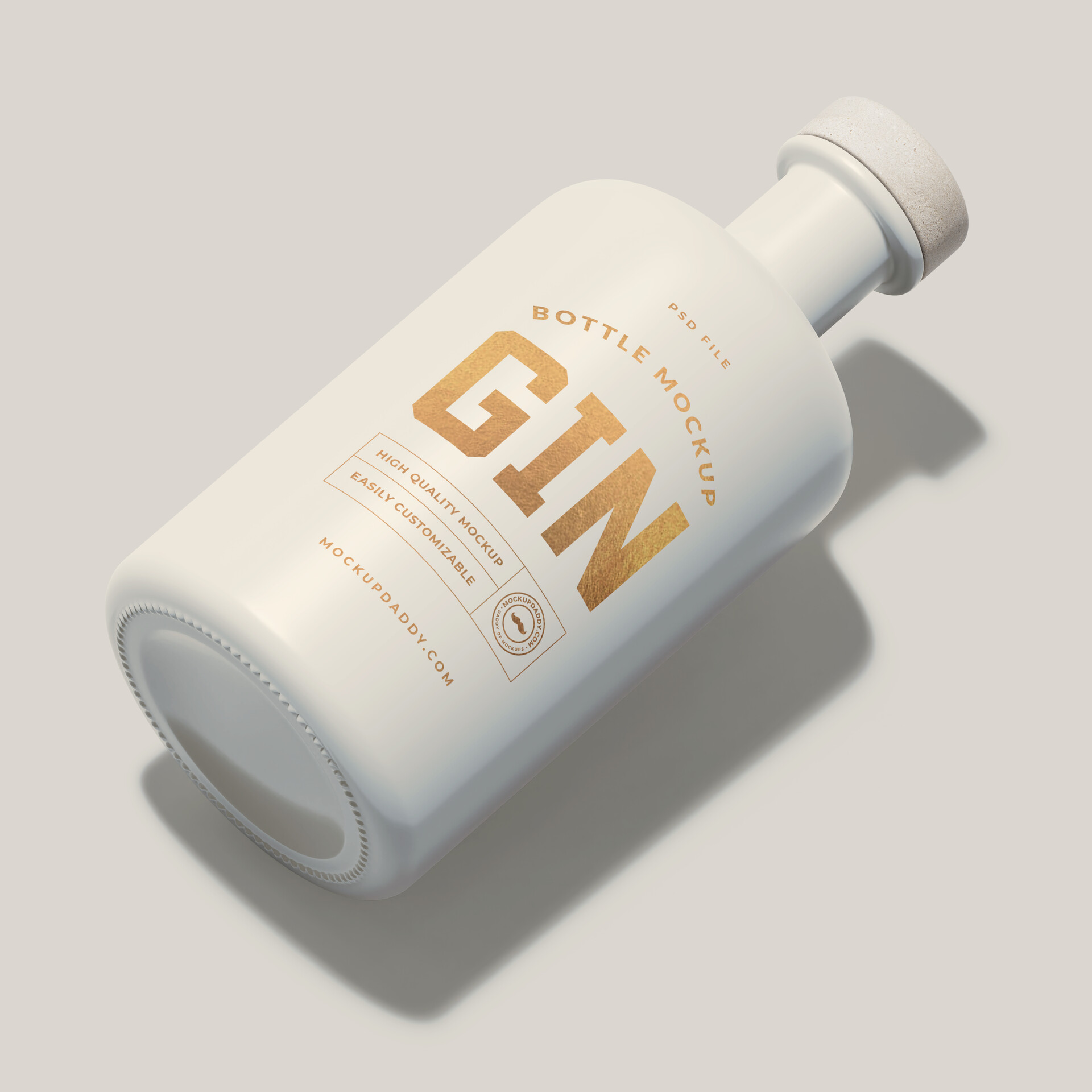The image features a highly detailed mock-up of a small to medium-sized white glass bottle with a screw-on cap. The bottle has the appearance of a photorealistic 3D render, indicated by the repeated word "mock-up." The background is a flat gray, providing a neutral canvas that highlights the bottle itself. The bottle, which could potentially be for gin, is adorned with gold lettering. At the top, it says "PSD File," followed by "Bottle Mock-Up Gin" in a stylized logo-type font. Below that, in a rectangular block, the text reads "High Quality Mock-Up, Easily Customizable." A circular logo featuring a mustache is also present, adding a touch of whimsy. Additionally, the phrase "mockupdaddy.com" is displayed both within the circle and at the bottom of the bottle. The scene is completed with a soft, impeccable shadow under the bottle, enhancing its realistic appearance.